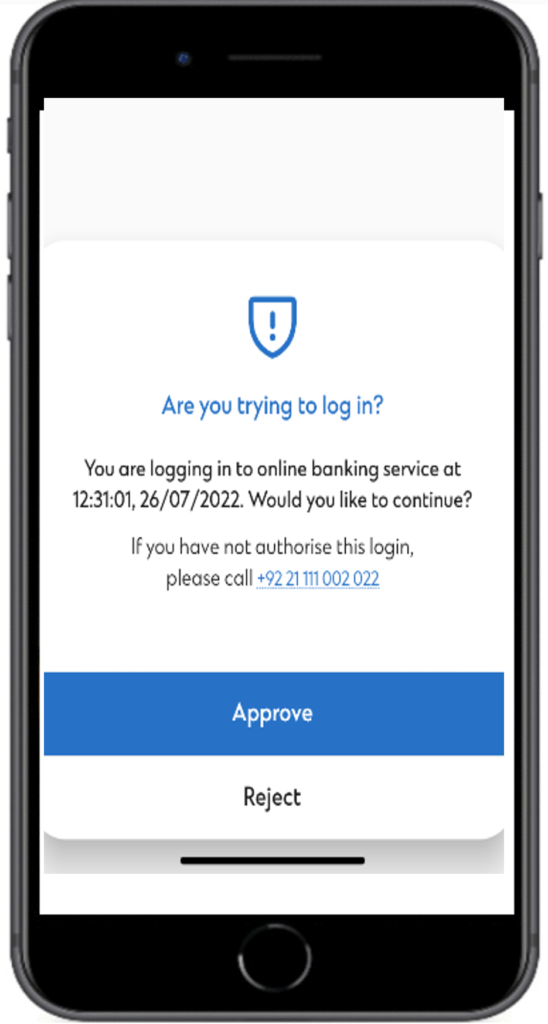A black smartphone with a black bezel is displayed against a white background. On the screen is a white pop-up notification featuring a blue shield icon with an exclamation mark inside it at the top. Below this icon, blue text reads, "Are you trying to log in?" 

The central portion of the notification contains black text stating: "You are logging in to online banking service at 12:31:01, 26-07-2022. Would you like to continue? If you have not authorized this login, please call +92.211.111.002.022." The phone number is highlighted in blue.

At the bottom of the notification are two buttons. The upper button is blue with white text that says, "Approve." The lower button is white with black text that says, "Reject." Additionally, a slider is visible at the bottom of the smartphone screen.